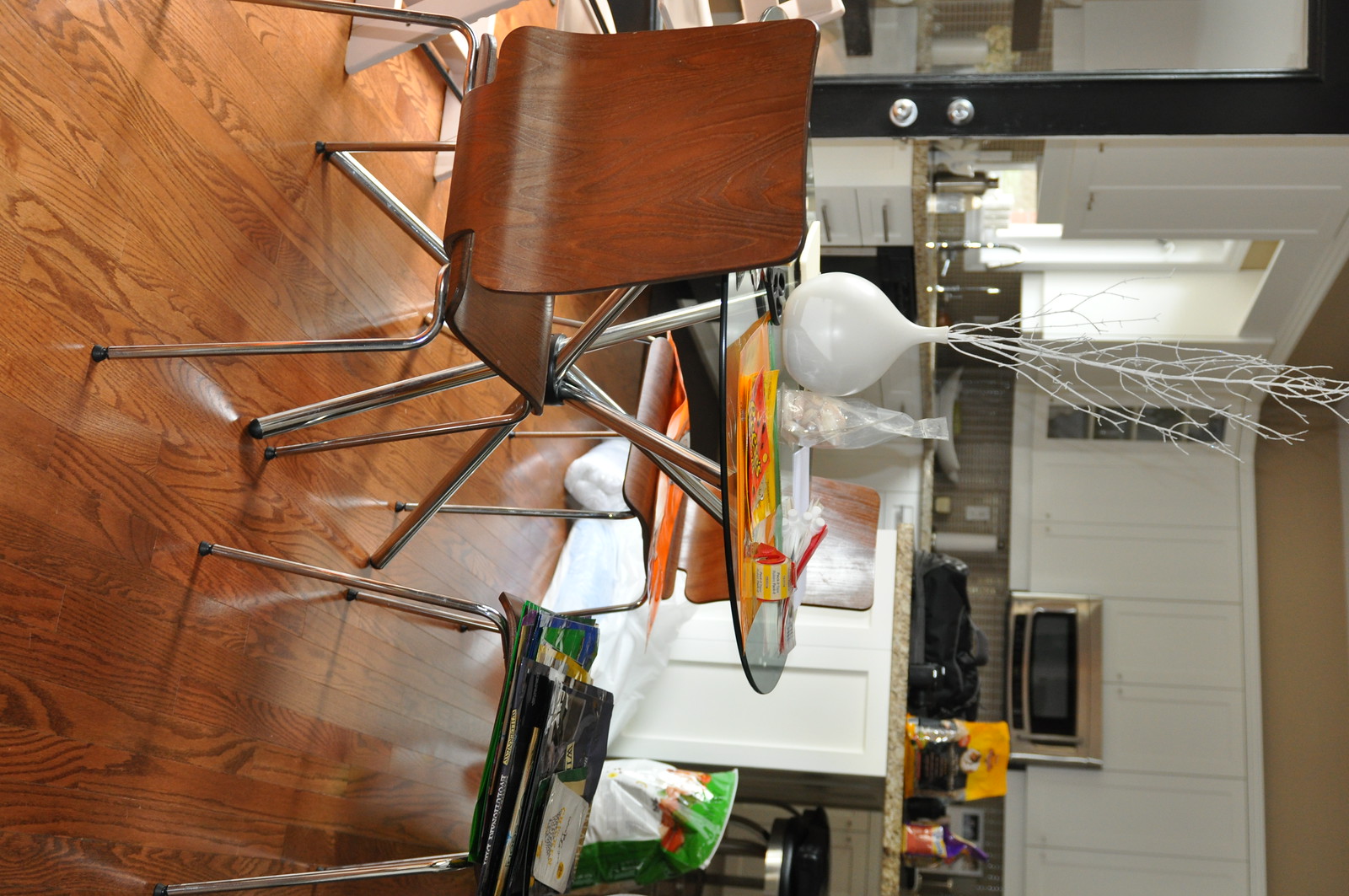A photograph taken with a 90-degree clockwise rotation captures a contemporary kitchen and dining area. To the left of the image, acting as the floor, lies a dark maple-colored wooden surface. Placed on the wooden floor is a round glass dining table with sleek aluminum or stainless steel silver legs. Accompanying the table is a modernistic wooden chair with matching aluminum legs, positioned nearby. Another chair is visible further to the right.

The ceiling, which appears at the bottom right corner due to the image's rotation, is a mustard-brown color. Just below the ceiling, wide white panels form part of the wall. An L-shaped kitchen counter, cluttered with various kitchen utensils, extends below the wall. The base of the counter consists of white cabinets.

At the center of the glass table sits a tear-shaped white porcelain vase, filled with long, spray-painted white tree branches. The table is also adorned with various clutter. Near the bottom of the image, which is technically the right-hand side when correctly oriented, there's a bag that appears to contain pet food, either for birds, dogs, or cats.